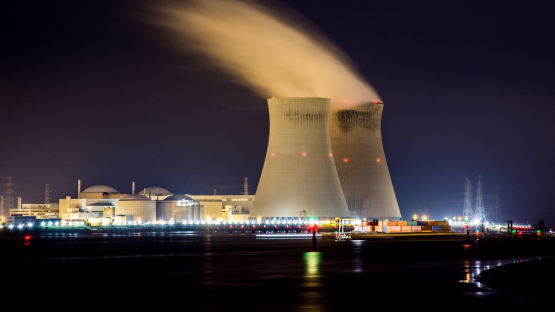This nighttime photo captures an expansive industrial complex, prominently featuring two towering structures reminiscent of nuclear reactors, each about 20 stories tall. These towers are grey and adorned with orange lights, releasing smoke or steam illuminated by additional lighting. The sky above is a deep, almost inky blue, devoid of clouds, and is subtly brightened by the myriad of lights from below. 

At the base of the towers, a series of smaller buildings and housing areas are clustered together, bathed in various lights—red, yellow, and white—that accentuate the scene. On the right, distant structures and tall scaffolding add to the depth of the complex. The bottom of the image is dominated by a dark, reflective surface that hints at the presence of water, capturing and mirroring some of the lights and shapes from above. The overall scene is a striking blend of industrial might and nocturnal tranquility, illuminated under the night sky.